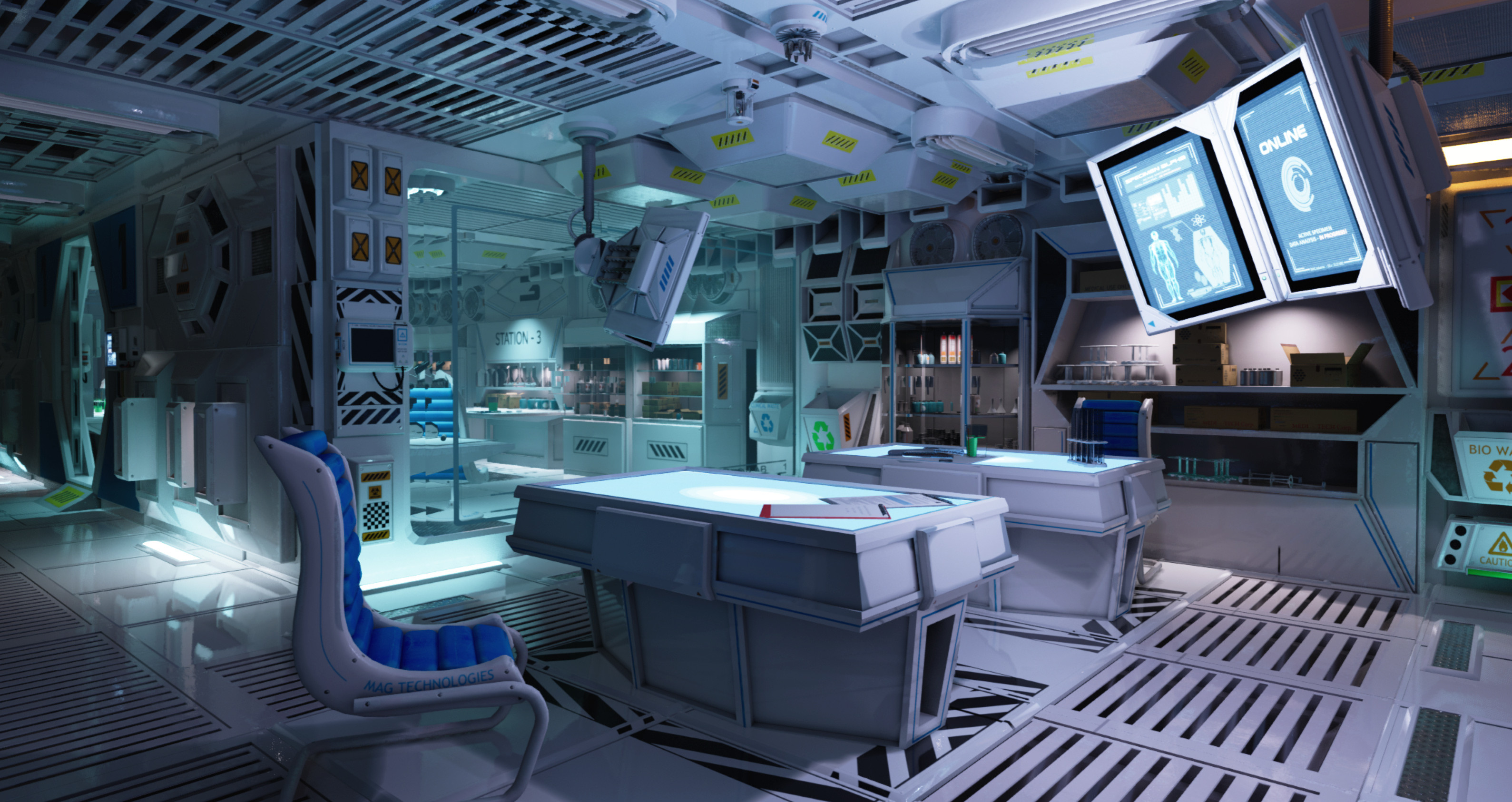The image depicts a highly futuristic command center that likely belongs to a digital or fictional environment, potentially from a video game. This spacious room is decked out in predominantly gray and white tones, with sleek, advanced equipment suggesting a high-tech operation. At the center are two gray tables with illuminated tops, accompanied by two gray chairs that feature blue cushions covering both the back and the seat. 

Facing the tables are two large monitors mounted on metal frames, displaying indistinguishable content but emanating a blue hue with white data and text. The ceiling is metal and features several metal containers affixed to it, while the floor is made of grating with visible gaps, possibly for drainage. Shelves and compartments line the room’s perimeter and a half-wall to the left of the desk area, each containing unidentified objects.

Additionally, there are multiple tablet-like devices, though currently they are not lit up, attached to the walls. On the far left, a hallway extends into darkness, and there’s a hatch or airlock, enhancing the impression of a spacecraft or advanced lab. The room’s meticulous organization and the presence of various technological apparatus contribute to its futuristic ambiance.